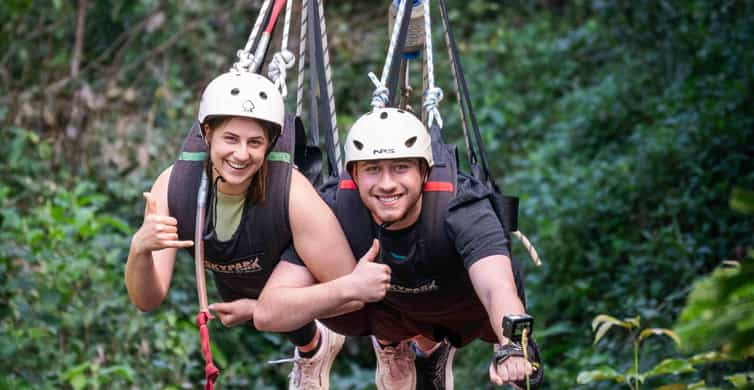This detailed color photograph features two individuals, a man and a woman, who appear to be hanging from a zipline amidst a lush, green jungle background. Both are equipped with white helmets; the man’s helmet showcases black "NRS" lettering, whereas the woman’s helmet bears a small black image resembling a cloud. They are suspended by black shoulder straps, which are distinctively marked with green bars for the woman and red stripes for the man. Each of them is held up by ropes that are light in color with darker stripes interwoven.

The man, positioned on the right, has a small camera attached to his left hand, presumably for capturing selfie videos, and his arm is interlaced around the woman. He is giving a thumbs-up gesture with his right hand and is dressed in a black shirt with tan-colored, thick, and leathery shoes. The woman, on the left, wears a green shirt underneath her gear and also tan-colored shoes. She is making a hang loose gesture with her right hand. Both individuals are smiling broadly, exuding confidence and pride in their adventurous activity. The verdant jungle, complete with thick foliage, serves as a picturesque backdrop.